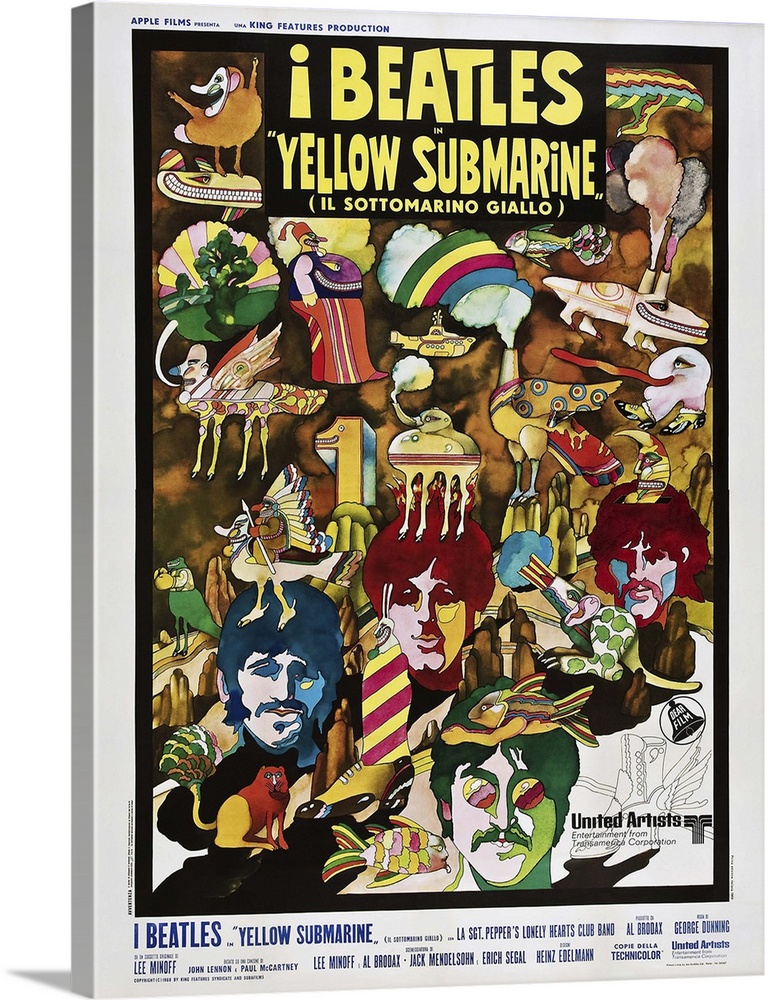The image is a highly artistic and colorful movie poster for "The Beatles: Yellow Submarine," with a distinctive white background featuring a black border. At the top left corner, the poster displays "Apple Films Presents" in a small font followed by "King Features Production." In bold yellow text at the very top, the title "The Beatles: Yellow Submarine" appears, along with the Italian subtitle "El Sotomarido Diablo." The central area of the poster is bursting with an array of vibrant and imaginative illustrations, including a whimsical yellow submarine, abstract figures, and fantastical creatures like a giant chicken, teapot-shaped birds, and other psychedelic elements. The characters, rendered in a sophisticated watercolor style, showcase bright greens, purples, yellows, and fuchsias. The bottom section of the poster features cartooned portraits of The Beatles from left to right. On the right-hand corner is the logo for United Artists. The very bottom of the poster lists the credits for the movie in blue text, providing details on the directors, designers, and other contributors. This striking design captures the essence of the film's creative and avant-garde spirit.